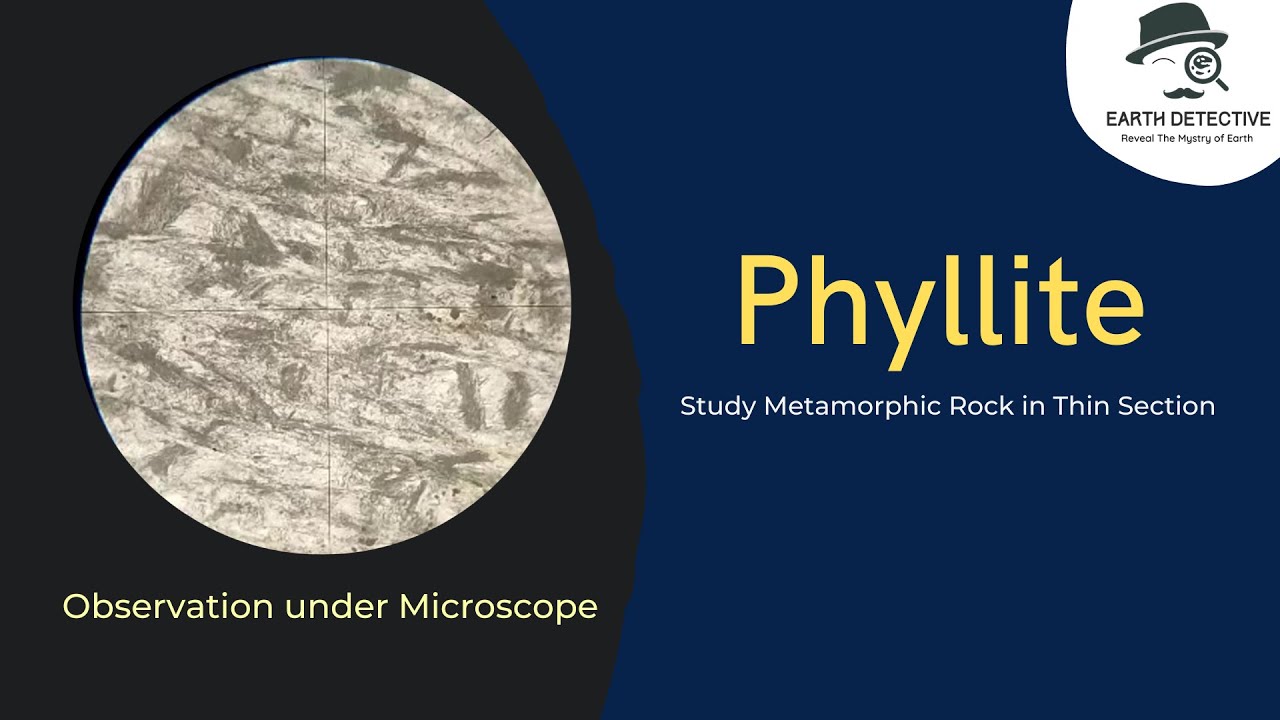The image is a rectangular illustration divided into two sections by a curved line. The left half features a black background with an off-white circular shape resembling a moon or marble with gray blobs. Below this circle, in clear text, it reads "Observation Under Microscope." The right half of the image has a dark blue background and prominently displays the text "Phyllite Study" in yellow, centered, with a subtitle underneath that reads "Study Metamorphic Rock in Thin Section." In the top right corner, within a three-quarter white circle, there's an illustration of a man wearing a black fedora, sporting a mustache, with his right eye closed and a magnifying glass held up to his left eye. Below this illustration, the text "Earth Detective" is visible, reinforcing the theme of investigation and research.